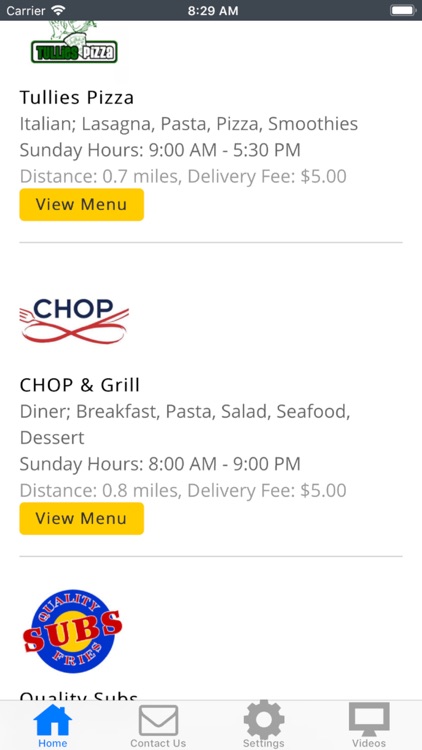The image appears to be a screenshot of a food-related application interface, displaying a list of various restaurants. The primary function of the app seems to be to help users find restaurants, potentially filtered by specific criteria such as dietary restrictions or cuisine preferences.

At the top of the list is "Thule's Pizza," which offers a variety of Italian dishes including lasagna, pasta, pizza, and smoothies. The restaurant operates on Sundays from 9:00 a.m. to 5:30 p.m., is located 0.7 miles away from the user, and has a delivery fee of $5. There is a prominently displayed "View Menu" button in yellow, allowing users to browse the restaurant's offerings further.

Following Thule's Pizza is "Chop and Grill," which features a diverse menu that includes diner-style items, breakfast, pasta, salad, seafood, and dessert. The Sunday hours for this restaurant align with the likely fact that the screenshot was taken on a Sunday. It is situated 0.8 miles from the user with a similar delivery fee of $5.

The third restaurant listed is "Quality Subs," but only the logo is visible, and no additional details can be discerned from the screenshot.

Overall, the image provides a clear presentation of three local dining options, emphasizing their cuisine types, distance, delivery fees, and operating hours specific to Sundays, aiding the user in making an informed dining choice.